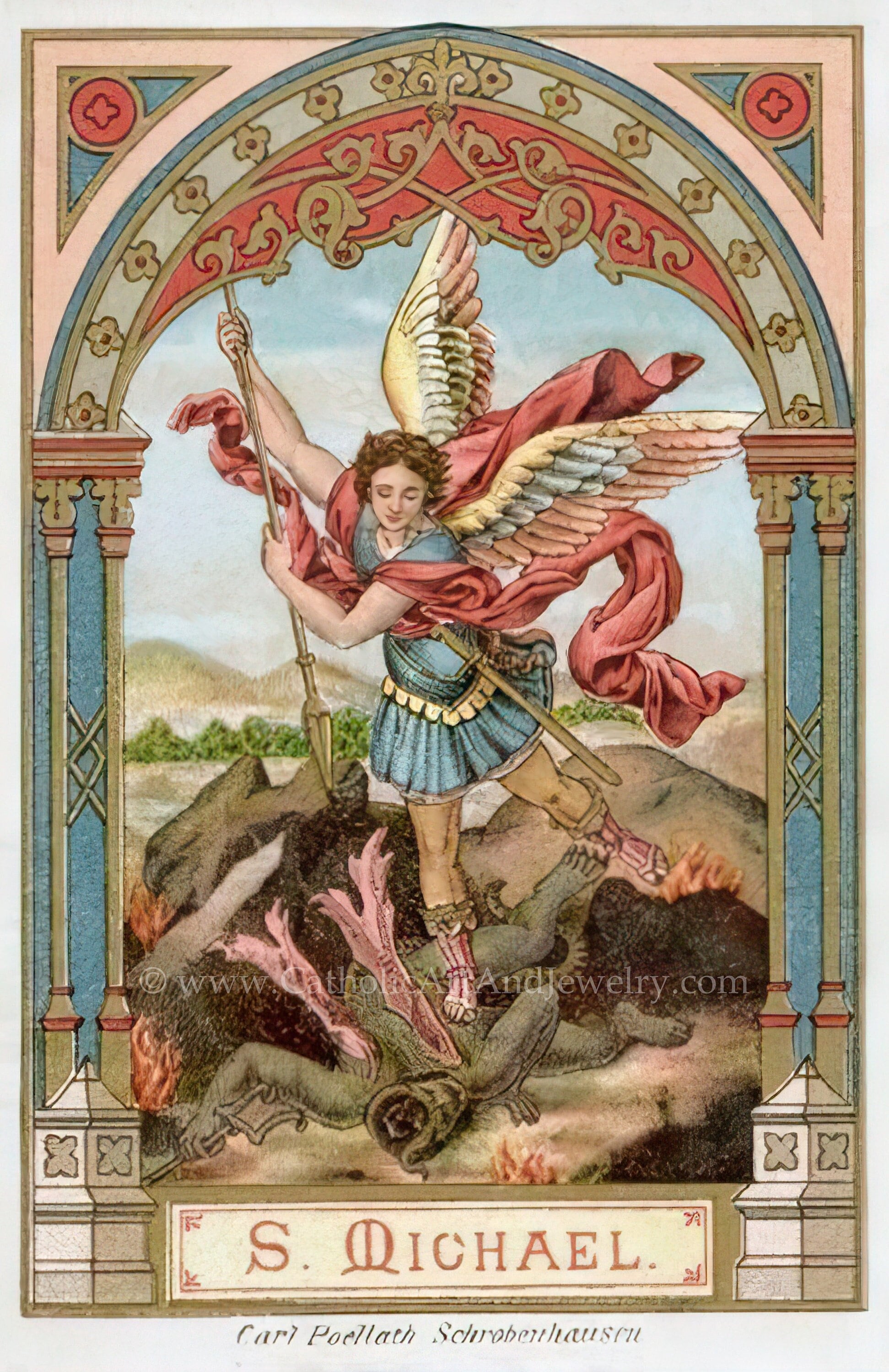The artwork is a rectangular piece with a thin grey border, in which the left and right sides are twice as long as the top and bottom sides. At the bottom of the border, in printed gold text, it reads "Karl Polath Schroenhausen," presumably the artist. A semi-transparent white watermark runs through the center, stating "copyright www.catholicartandjewery.com." The scene is of an angel with wings, wearing a blue tunic and pink sandals, about to stab a grey demon with red wings using a large gold spear. The angel stands atop the demon, symbolizing victory. The background features elements reminiscent of royal architecture, with gold and beige arcs, fancy structures, and pillars. Additionally, the backdrop includes a natural landscape with blue skies, hills, mountains, trees, plants, water bodies, and fire. There are green and black elements on the demon, and the angel also has a sword hanging from a waist belt in a scabbard. The artwork blends classical and natural elements, creating a richly detailed and dynamic scene.